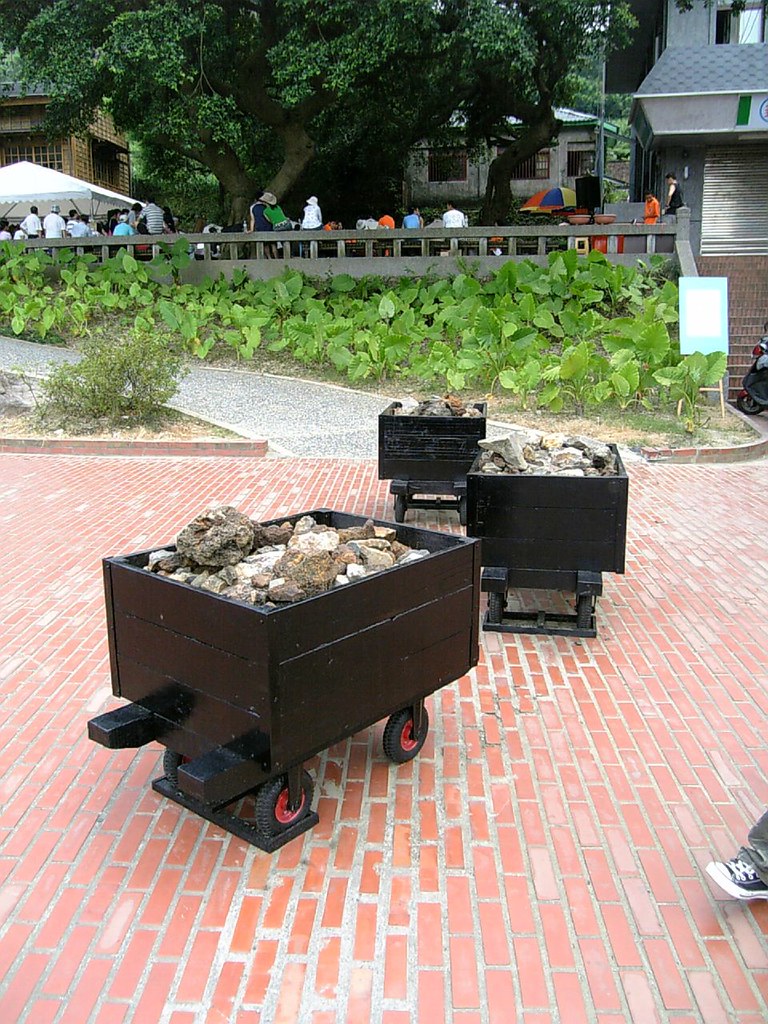In this color photograph, taken outdoors during the day, we see three dark-colored carts, most likely painted in either very dark brown or black, positioned in a neat row extending away from the camera on a red brick pathway, which could be a driveway or entryway. Each cart is mounted on four wheels, equipped with locks, and filled with various sizes of broken concrete or rocks. The carts, which resemble small train cars or large wheelbarrows, are not attached to any visible towing mechanism.

On the right edge of the photo, a partial sneaker of a person is visible. The brick pathway is adjacent to a gravel path that leads off the frame, surrounded by greenery. In the background, slightly elevated above the path's level, is a lively gathering in what appears to be a restaurant patio. The patio features multiple seating areas under a white gazebo-like tent and a colorful rainbow umbrella. Scattered plants act as a buffer between the carts and the seated people enjoying the event. A large tree provides shade to the gathering, contributing to the festive, outdoor atmosphere.